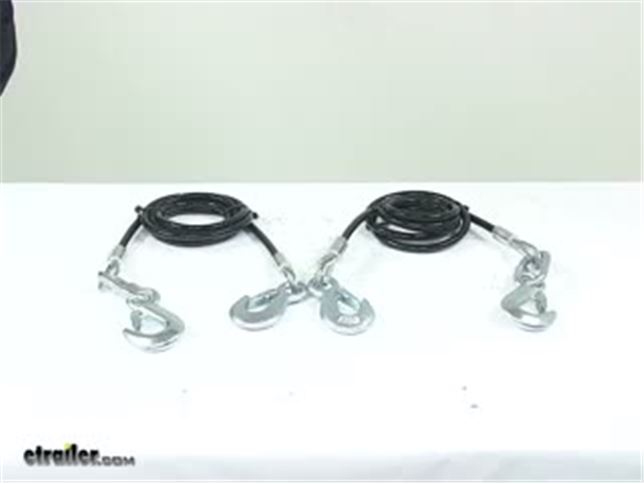The image depicts two bunches of black cords or wires, each featuring a pair of silver carabiner-style hooks on their ends. These cords are arranged side by side on a white tablecloth that covers a table. The cords, possibly coaxial, are looped into circular shapes with their hooks prominently displayed. The background consists of a green wallpaper, providing a stark contrast to the white tablecloth and black cords. In the bottom left corner of the image, partially obscured but readable, is the text "ctrailer.com". Additionally, a black sleeve, likely belonging to a person, intrudes slightly into the frame from the top left corner, indicating the presence of someone nearby.